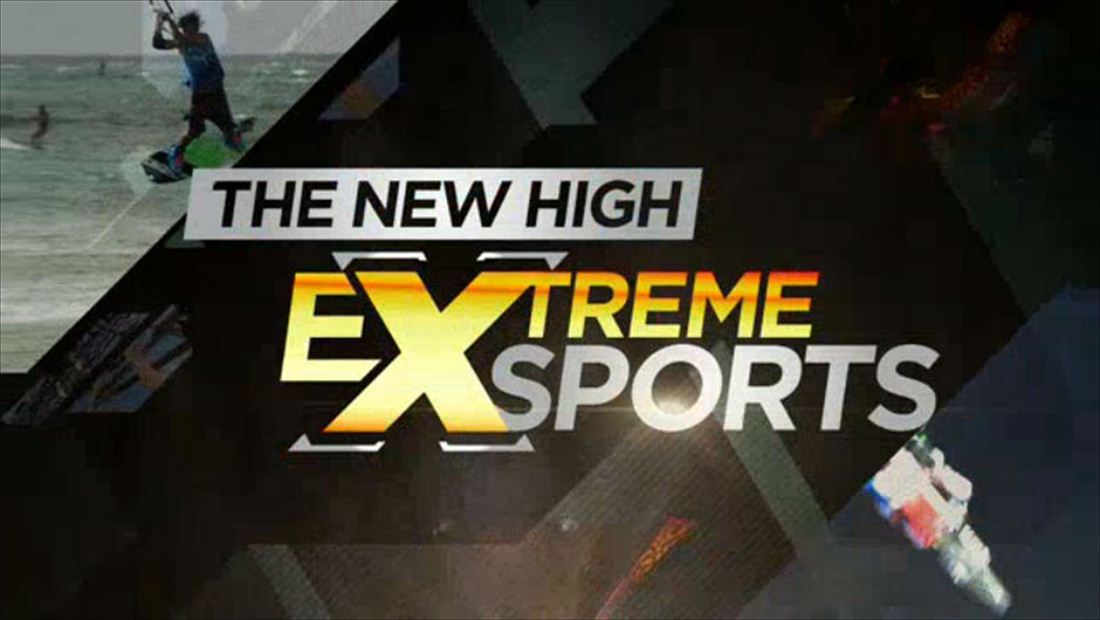The image prominently features a dark and dramatic background. In the top left corner, a vivid action shot captures men engaging in an extreme water sport, possibly water skiing or boarding, with muted green water and a gray sky enhancing the intensity. The main focal point of the image, however, is the bold text occupying most of the space. At the top, "LIEU HAI" is displayed in black capital letters on a grey slightly-parallelogram background. Below it, the word "EXTREME" is presented in large, yellow, capitalized letters with a red stripe running through them; the "X" is significantly oversized and accented with silver caps at each end. Beneath this, the word "SPARKS" (or "SPORTS," based on varied interpretations from the sources) appears in a greyish white or silver hue, also in capital letters. The lower right portion of the image is dark gray, and there's an indistinct image, predominantly white with some red and blue elements, possibly indicating further action or devices related to the extreme sport. Overall, the image strikes a balance between intense visual action and striking textual elements, resembling a high-impact advertisement.